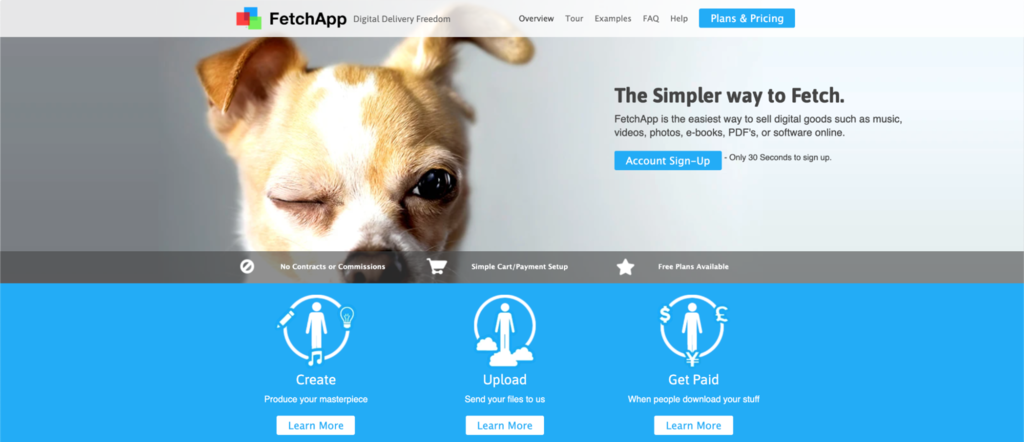In the upper section of the website, the background is a translucent white, allowing a subtle glimpse of a dog's ears. This dog, depicted in the middle section, appears to be a chihuahua, predominantly brown with a blue middle section, one eye open and the other closed, showcasing its expressive black eyes.

The layout contains three vertically aligned squares on the left side, progressing in size from top to bottom: the top square is red, the middle one is green, and the bottom square is blue. Bold black text reading "Fetch App" is positioned prominently, followed by the tagline in regular black text, "Digital Delivery Freedom." Navigation options include "Overview" (highlighted in a darker shade to indicate the current section), "Tour," "Examples," "FAQ" (Frequently Asked Questions), and "Help."

A blue rectangular button labeled "Plans" with a white 'N' symbol is prominently featured. The background transitions to gray as the description shift focuses to the selling proposition of Fetch App, emphasized by the phrase "Fetch App is the easiest way to sell digital goods such as music, videos, photos, eBooks, PDFs, or software online." Further down, another blue rectangle contains "Account Sign Up" in white text, with an additional note in black proclaiming "Only 30 Seconds to Sign Up."

At the bottom, a gray-bordered section lists features in white text: "No Contracts or Commissions, Simple Contract Payment Setup, Free Plans Available as well." Below this, a trio of blue buttons, each labeled in white, provides options to "Learn More" about getting paid, uploading files, and producing a masterpiece.